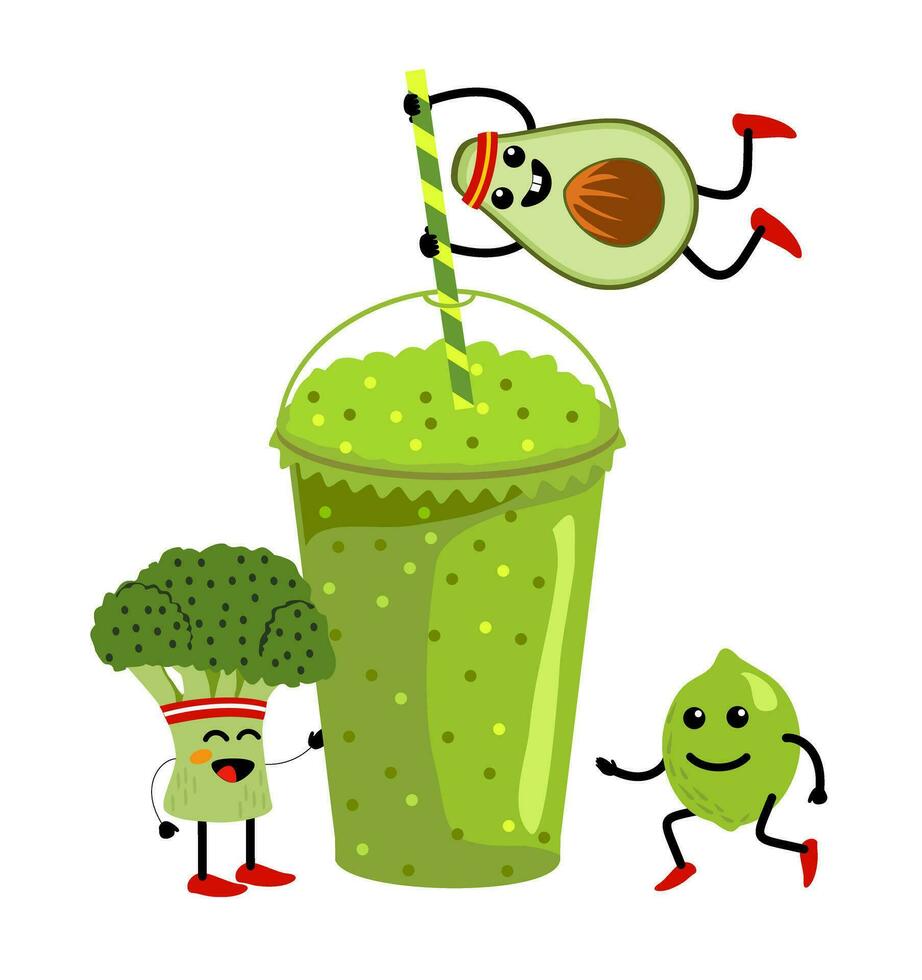This vibrant illustration depicts a lively green smoothie in a clear plastic cup with a domed lid and a two-tone green striped straw. The smoothie itself is a vivid green, interspersed with light and dark green polka dots. Adding a playful character to the scene, a cheerful half-avocado with a brown seed in its center is hanging horizontally from the top of the straw. The avocado sports a yellow and red striped headband, red shoes, and exhibits a big smile with two prominent buck teeth.

To the left of the smoothie cup, a friendly piece of broccoli leans against the cup. This broccoli character is outfitted with a red and white striped headband, red shoes, and a joyous smile, complete with red cheeks and closed eyes. On the right side of the cup, a happy lime, also wearing red shoes, appears to be either running or dancing. This lime character has black eyes and a broad smile. Together, these endearing caricatures of healthy greens bring an energetic and wholesome vibe to the illustration.